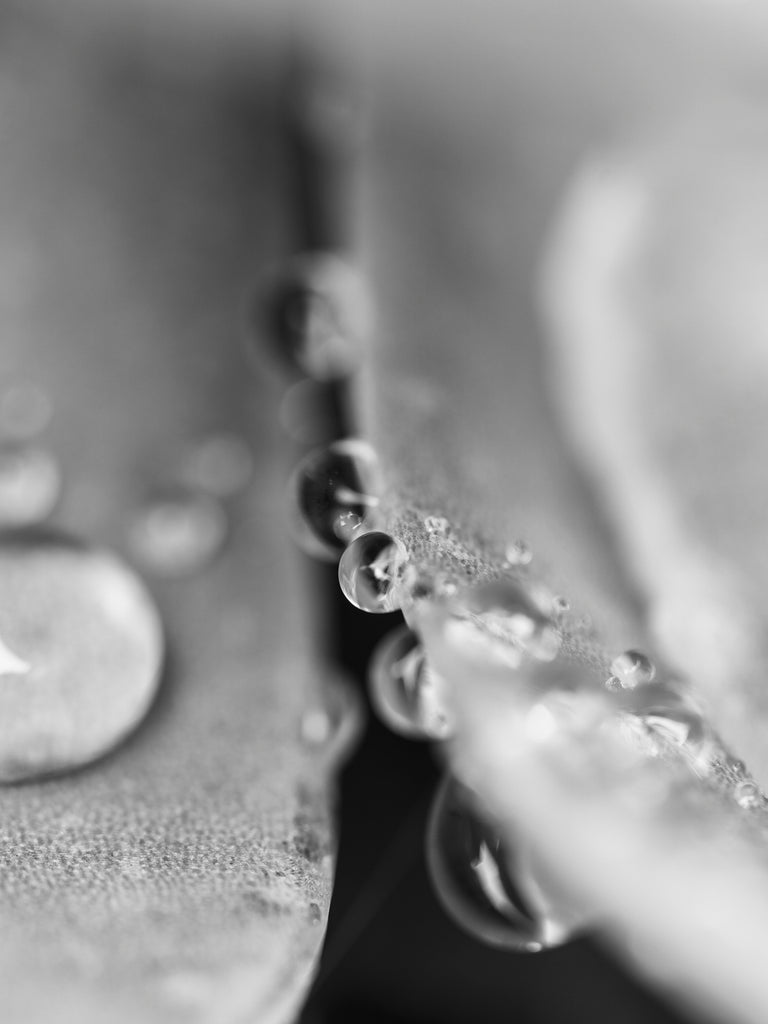This image features a highly detailed, black and white close-up of numerous water droplets on a leaf, with the photo taken in a gray, monochrome scheme. The droplets, varying in size from very tiny to quite large, are dispersed across the surface of the leaf, exhibiting a mixture of textures and opacities. Some droplets are oriented upwards, others downwards or to the sides, creating a dynamic scene. The background is predominantly black, adding contrast to the grayish tones of the leaf and water droplets. The top and the bottom right corner of the image are slightly blurred, enhancing the focus on the central droplets. The leaf itself shows texture through a pattern of white and black dots. Despite the lack of color, the photo reveals significant details, such as shadowed black tops and lighter bottoms on the droplets, suggesting depth and translucence. Some droplets appear to pool more on one side of the leaf, while others rest delicately on its surface.